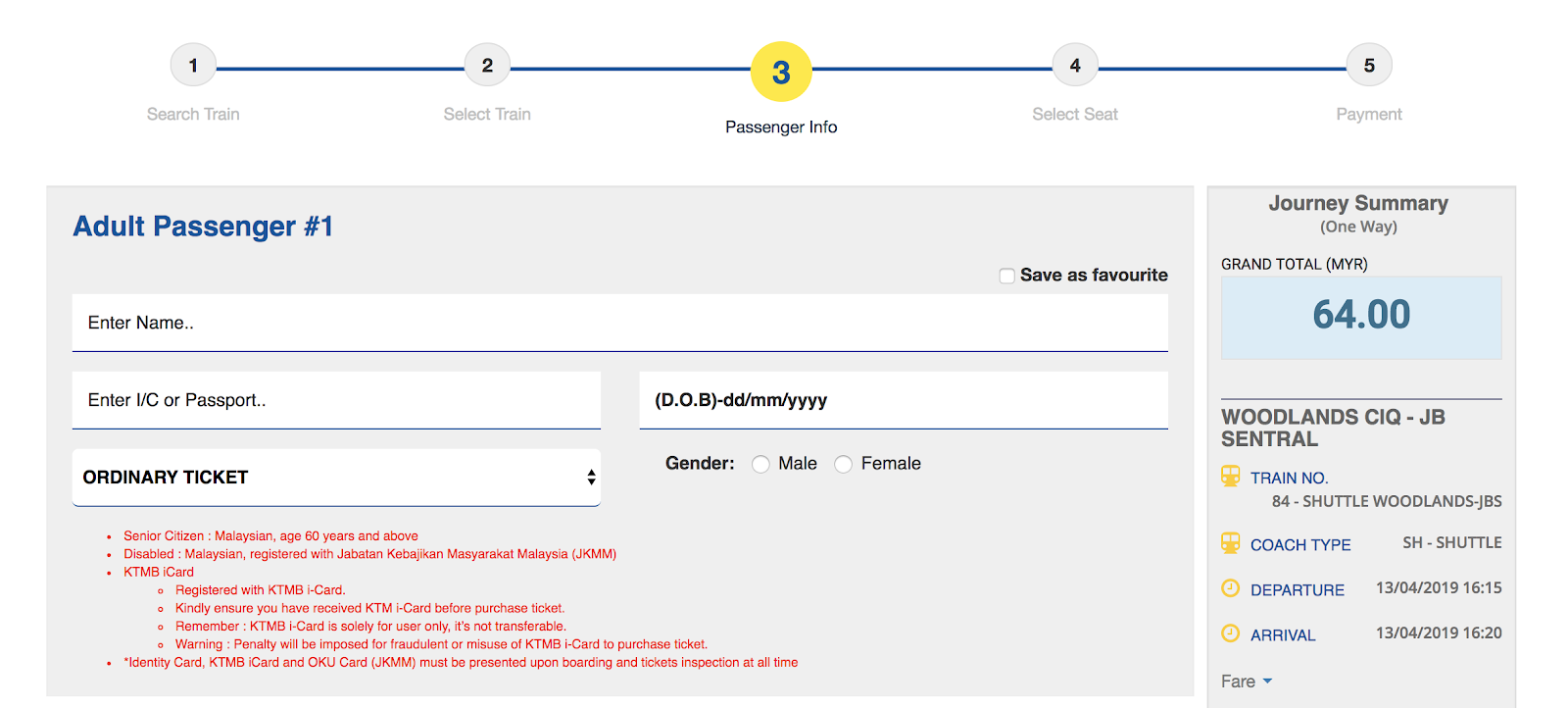This screenshot captures the third step of a five-step train booking process on a transportation website. At the top of the screen, a numbered progress bar from 1 to 5 visually indicates the stages of the booking procedure. The steps are labeled as follows: 1) Search Train, 2) Select Train, 3) Passenger Info (highlighted in yellow to show the current step), 4) Confirm, and 5) Payment. 

The user has already completed the "Search Train" and "Select Train" stages. They are now entering mandatory passenger details like name, passport number, date of birth, ticket type, and gender. The left side of the screen lists these steps, while fields for personal information occupy the central section.

To the right, a blue box prominently displays the number "64," representing the total cost of the train ride in the selected currency.